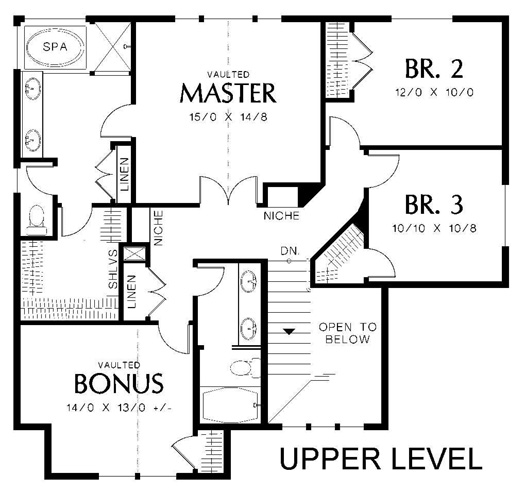This detailed blueprint of a house's upper level, set against a white background, features several distinct rooms and areas. In the bottom right corner, the blueprint is labeled "Upper Level." Starting from the entrance, a staircase is positioned to the left. Beyond that, to the right of the entry, an open area is marked "Open to Below."

Continuing straight leads to Bedroom 3, measuring 10 feet 10 inches by 10 feet 8 inches. If you proceed further, you'll arrive at Bedroom 2, sized at 12 feet 0 inches by 10 feet 0 inches. Returning to the hallway and turning to the right, you enter the "Vaulted Master" bedroom with dimensions of 15 feet 0 inches by 14 feet 8 inches. To the left inside the master bedroom, there is an adjoining bathroom containing a spa, a linen closet, and an additional room surrounded by shelves.

Exiting the master bedroom and turning right once again, you'll find another bathroom to the left and a linen closet to the right. If you proceed straight ahead, you will reach a room labeled "Vaulted Bonus," measuring 14 feet 0 inches by 13 feet 0 inches.